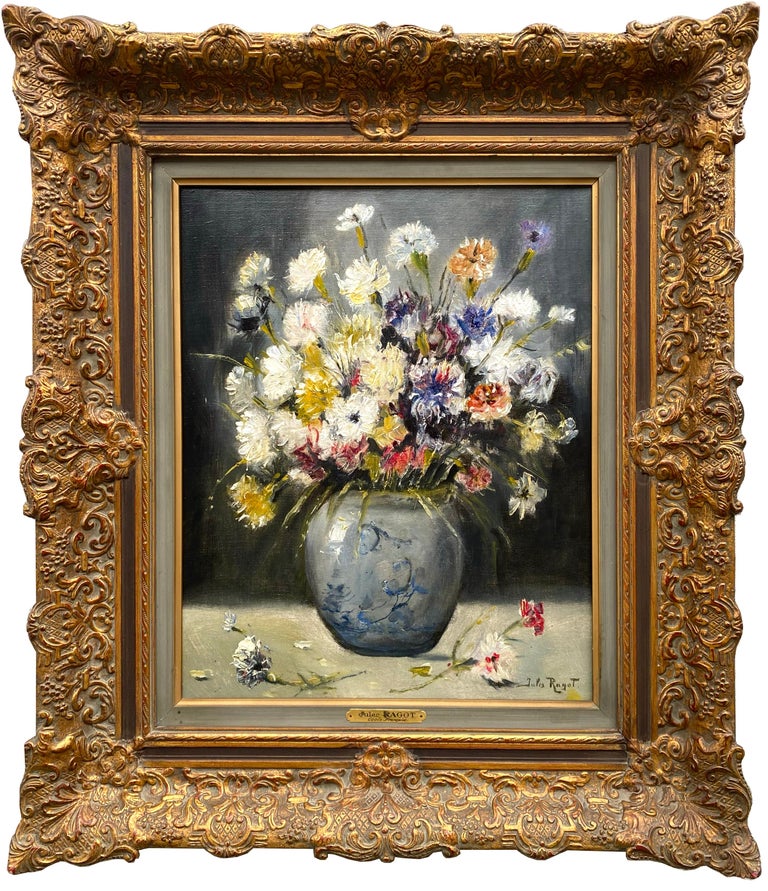This image showcases an ornate painting framed in an antique, bronzy-gold, or dark gold frame with intricate and elaborate designs, including swirls and ridges that raise up into points at all four sides. The frame is notably wide, approximately three to four inches. Inside the frame, the painting features a blue and gray vase with various wildflowers, prominently displayed on a light-colored table. The vase is round and stout, filled with flowers that reach the top of the painting. The flowers exhibit a vibrant array of colors, including whites, deep blues, pinks, reds, yellows, oranges, and purples, resembling daisies and carnations. A few flowers have fallen from the bouquet and lie scattered around the vase. The background of the painting consists of light gray and blue hues, with hints of green at the bottom. The artist's signature is located at the bottom right of the painting, and there is a decorative label in gold with black lettering at the bottom of the frame, though its text is not clearly visible.